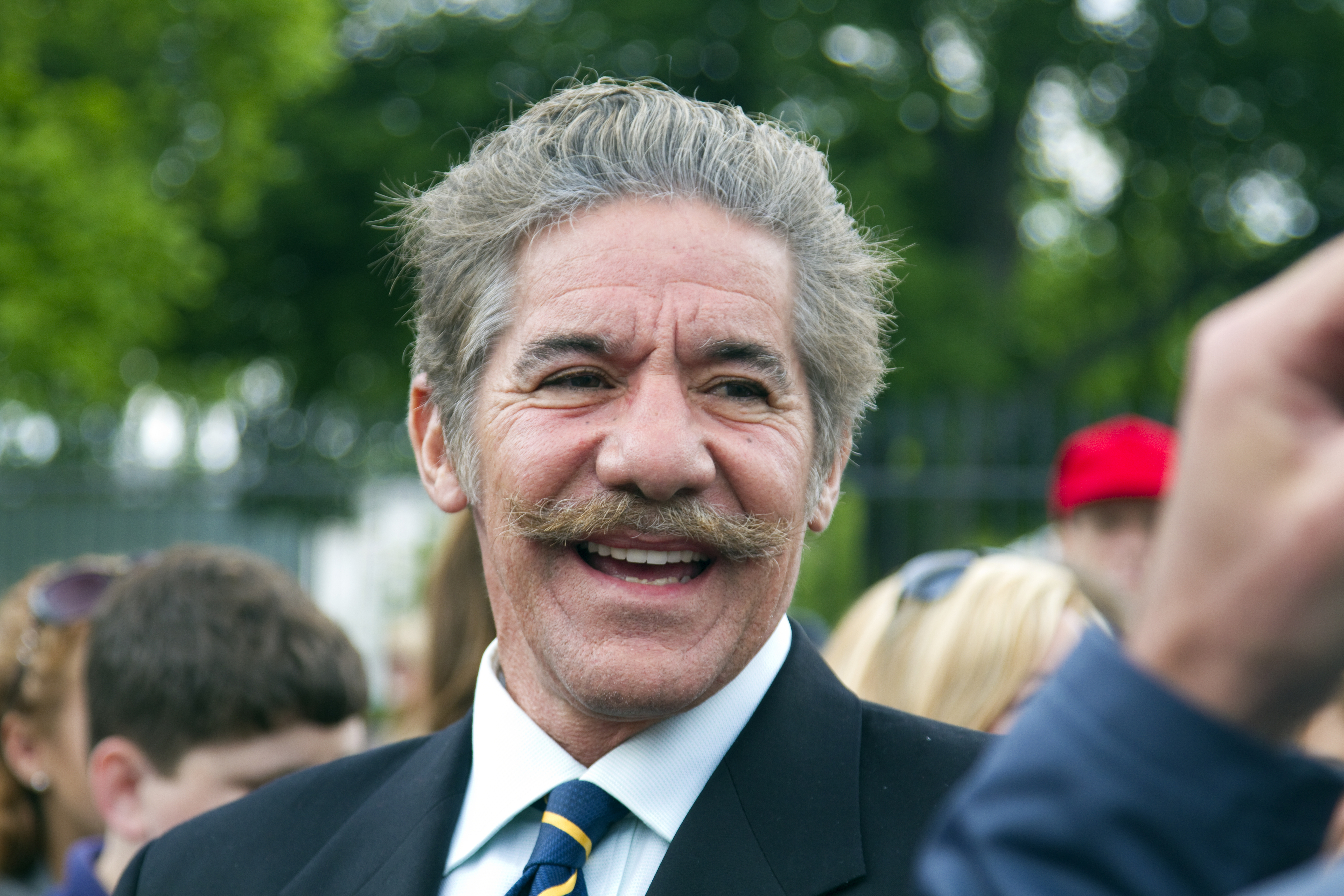This landscape-oriented color photograph features Geraldo Rivera, a distinguished older man with a distinctive appearance, standing slightly left of center and viewed from his head to mid-chest. Rivera is characterized by his slicked-back gray hair, prominent handlebar mustache that's a mix of brown and gray, large bulbous nose, dark eyes, and bushy eyebrows. His mouth is open in a toothy smile, and he seems to be engaging in conversation with someone off-frame, indicated by the visible yet blurry back of a hand on the right side of the image. Rivera is dressed in a dark blue blazer, white shirt, and a blue tie with yellow stripes.

The background is populated with several indistinct figures, including a blonde-haired person, a young child with short brown hair, women, and a man with a red hat. Their faces are not clearly visible, mostly presenting just the tops of their heads. Beyond these figures, the scene includes a blurry fence and out-of-focus green trees, suggesting an outdoor setting. The photograph employs a style of representational realism, capturing a candid moment of Rivera amid a crowd.